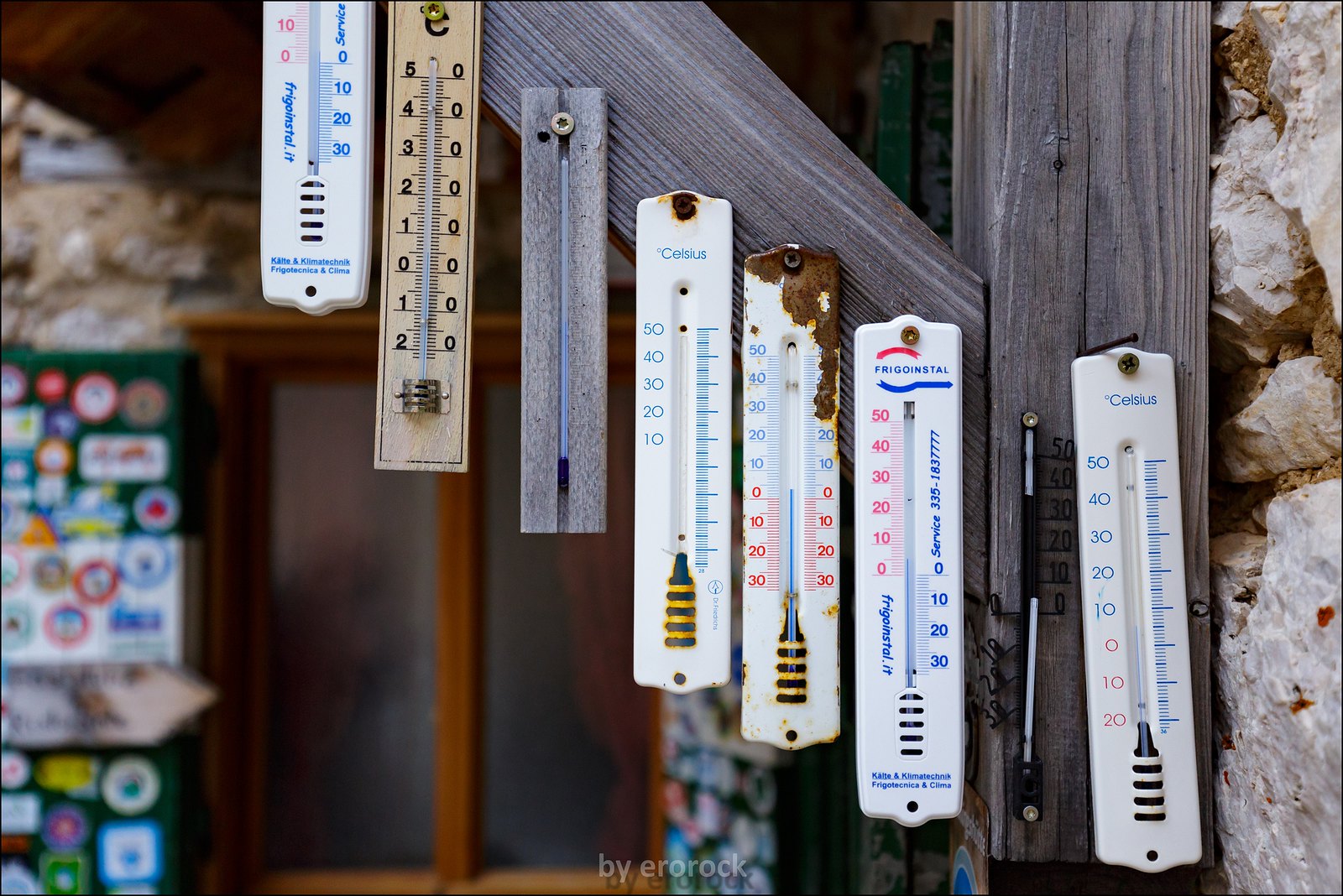A series of thermometers are mounted on an aged and weathered wooden beam supported by a wooden brace. The majority of the thermometers are affixed to the support, while two are attached directly to the beam. Most thermometers are secured with screws, and there's an errant nail positioned above one, but not through it. In the lower backside to the left, a green board featuring several circles with multicolored borders—orange, red, blue, and green—is partially visible, though too blurry to discern specific details. The backdrop consists of a stone wall, and to the right, partially visible, is either a cabinet or a window with light brown frames and red curtains.

The wooden beam itself is dark brown, noticeably weathered, old, and unfinished. Adjacent to the beam is more of the stone wall, and some unidentified green wood visible behind it. The thermometers are of various designs and sizes, arranged in a diagonal descending pattern from the upper left to the lower right along the support beam.

From top to bottom:
1. The upper-left thermometer is white with blue numbers on the right and red numbers on the left. The accompanying text is too blurry to read.
2. Below it, a light brown thermometer with black numbers ranging from 5 at the top to -2 at the bottom, though it lacks the negative symbol.
3. The third appears to be an unmarked wooden piece with a glass rod inside, featuring dark blue coloring at the bottom.
4. The fourth and fifth thermometers have similarities but are not identical. The first of these is white with blue numbers ranging from 50 to 10 and has a small scale on the right with a yellow and green striped bottom. The second of these has significant rust in the upper right, blue numbers from 50 to 10 on the left, red numbers from 0 to -30 below, and a yellow and brown striped bottom.
5. Next is a thermometer with red numbers from 50 to 0 on the left and 0 to 30 on the right, with unreadable small text and blue and white stripes at the bottom.
6. Following that, a barely visible thin thermometer with a black backing and white rods on both ends, black numbers from 50 to 0 on the left on the wood, and slanted, barely visible numbers from 0 to 30 on the left side.
7. The last visible thermometer is white with blue numbers from 50 to 10 on the left and red numbers from 0 to -20 below. It features a blue scale on the right and black and white stripes at the bottom.